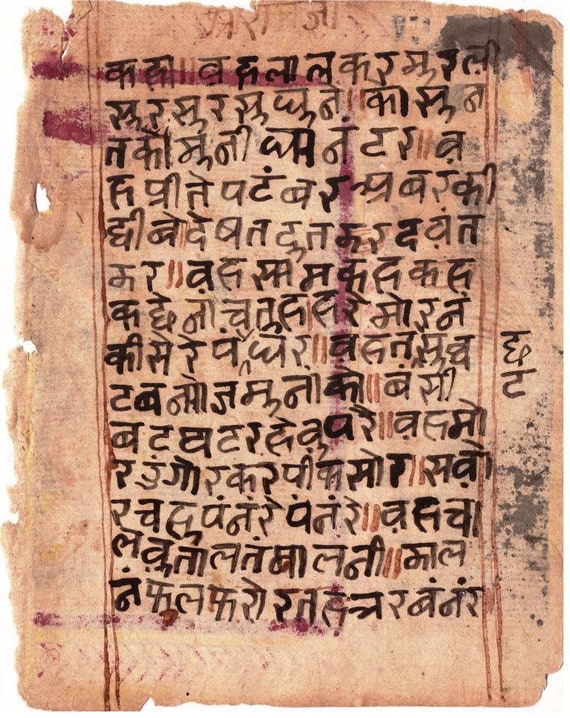This image depicts a photograph of an ancient, weathered page, possibly originating from a scroll or manuscript. The page is composed of a ragged, parchment-like material with tattered edges and a pale, pinkish-yellow hue, indicative of significant aging and exposure. The page is filled with rows of handwritten text in an unknown ancient script, possibly Sanskrit, though its exact nature remains unidentified. 

Hand-drawn double reddish-brown lines frame the text, forming margins about an inch from the left and right edges, which also highlight the presence of a preserved writing space in the center. The margins and text are detailed with black ink markings, some of which appear faded, suggesting water damage or extensive use. Additional smudges and marks, including an elongated U-shaped red smudge and spots of what could be mold or mildew, are visible, adding to the historical character of the document. Various tears and holes are evident along the frayed left side and the top edge, while the right and bottom edges, though aged, remain relatively intact. This detailed observation underscores the document's considerable antiquity and the fragility of its material form.